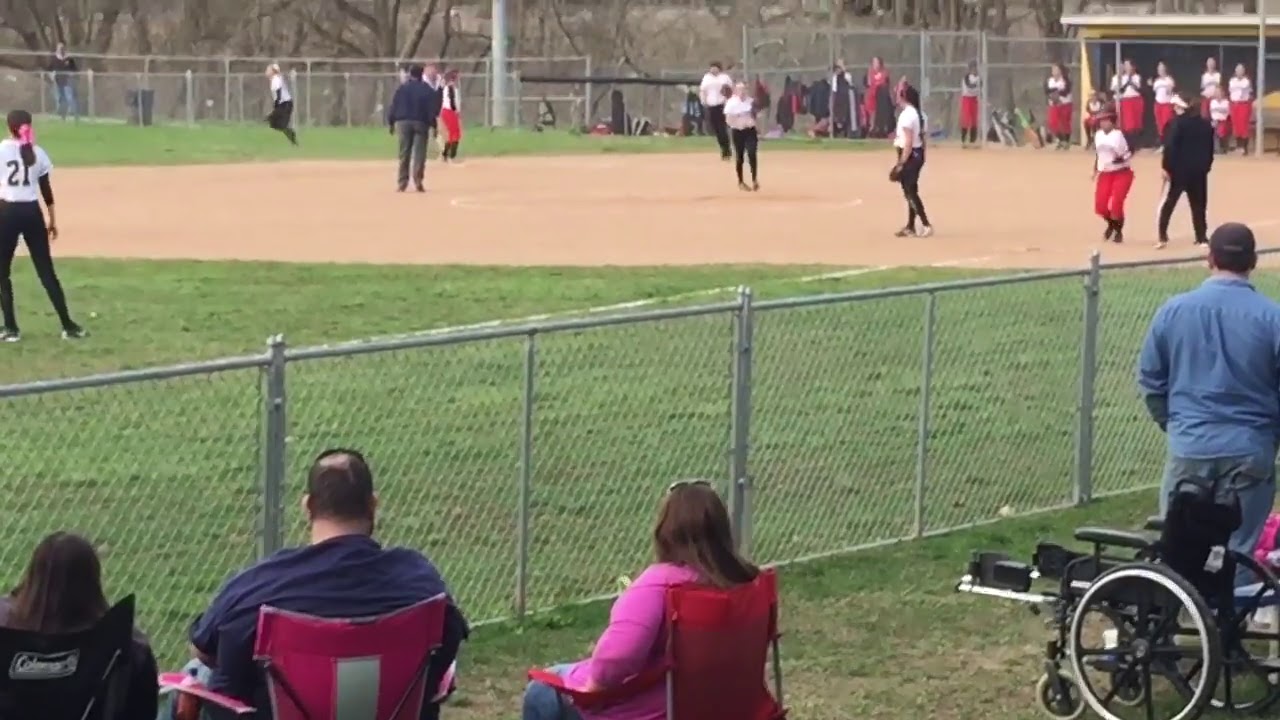The detailed image captures a high school or middle school girls' softball game, set on a gloomy, overcast day. The scene is framed by a chain-link metal fence, capturing a mix of brown dirt and green grass patches on the playing field. The players, mostly in the age range of teenage girls, are divided into two teams. One team is dressed in white shirts paired with black pants, while the opposing team sports white shirts and red pants. The game action includes a player on third base and another on first base, with an umpire interacting on the field. In the upper left, the dugout is visible, populated with team members in white shirts and red pants.

The spectators, positioned along the sidelines and slightly to the right of the field, include three adults seated in a mix of sports chairs—two red and one black—and at least one person in a wheelchair. Autumnal trees with no leaves serve as the backdrop, reinforcing the fall setting. The colors captured in the scene include brown, green, white, black, red, yellow, blue, silver, and gray, adding richness to the composition of this photograph taken from the audience's perspective.